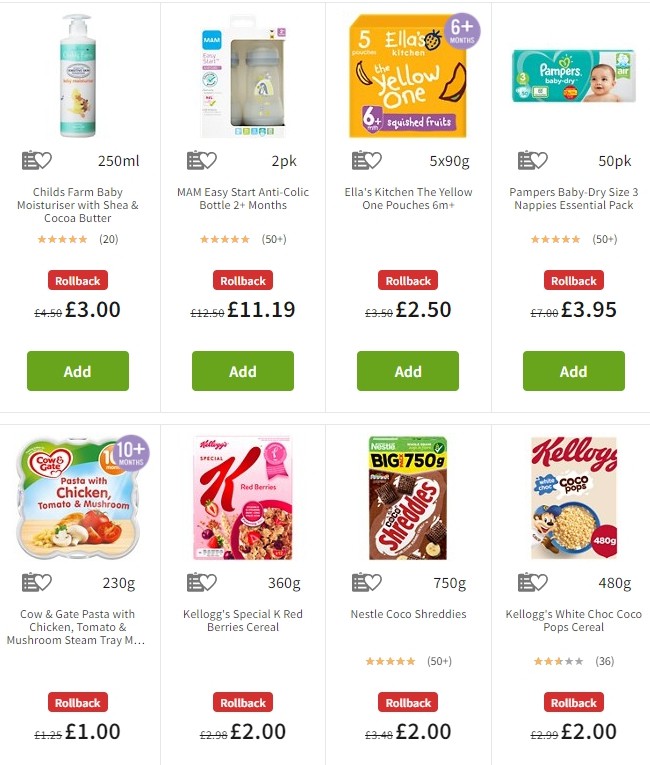The image is a screenshot from a shopping website featuring a selection of eight baby and grocery products arranged in two rows. 

In the top row, from left to right:
1. A blue bottle of baby moisturizer.
2. An anti-colic baby bottle.
3. A yellow pouch of Ella’s Kitchen baby food.
4. A box of Pampers Baby Dry Size 3 nappies (Essential Pack).

In the bottom row, from left to right:
1. Cow & Gate pasta with chicken, tomato, and mushroom steam tray.
2. A box of Kellogg’s Special K Red Berries cereal.
3. A box of Nestle Cocoa Shreddies cereal.
4. A box of Kellogg’s White Choco Pops cereal.

Each item features a red alert banner below it indicating a "Rollback" price, with the price listed in British pounds beneath the banner. The website source is not specified in the image.